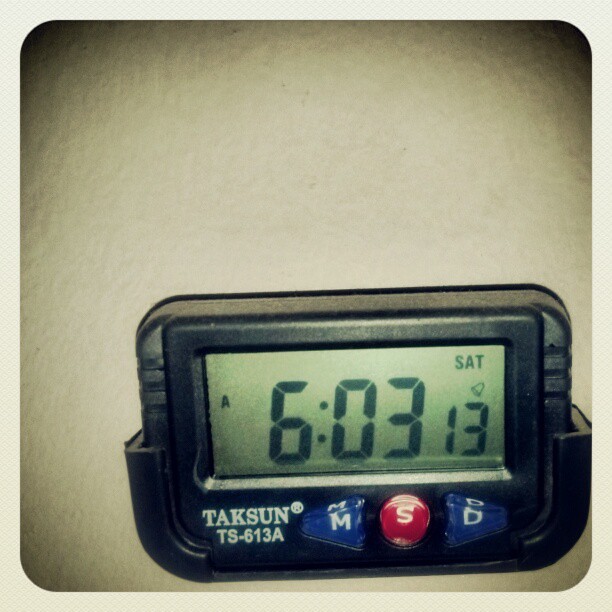In this image, the primary focus is on an electronic timer positioned in the bottom right-hand corner against a white wall backdrop. The wall features subtle shadows radiating from each corner, adding depth to the scene. The image edges are softened with an off-white border and rounded corners, giving it a refined appearance. The timer itself is encased in a sleek black frame, with the brand name "TACSON TS-6138" visibly inscribed on the bottom. The control interface includes three distinct buttons: a blue arrow button marked with a white "M," a round red button labeled "S," and a blue triangle button with a "D" pointing to the right. The digital display of the timer shows the time as "6:03" and indicates that it is Saturday.